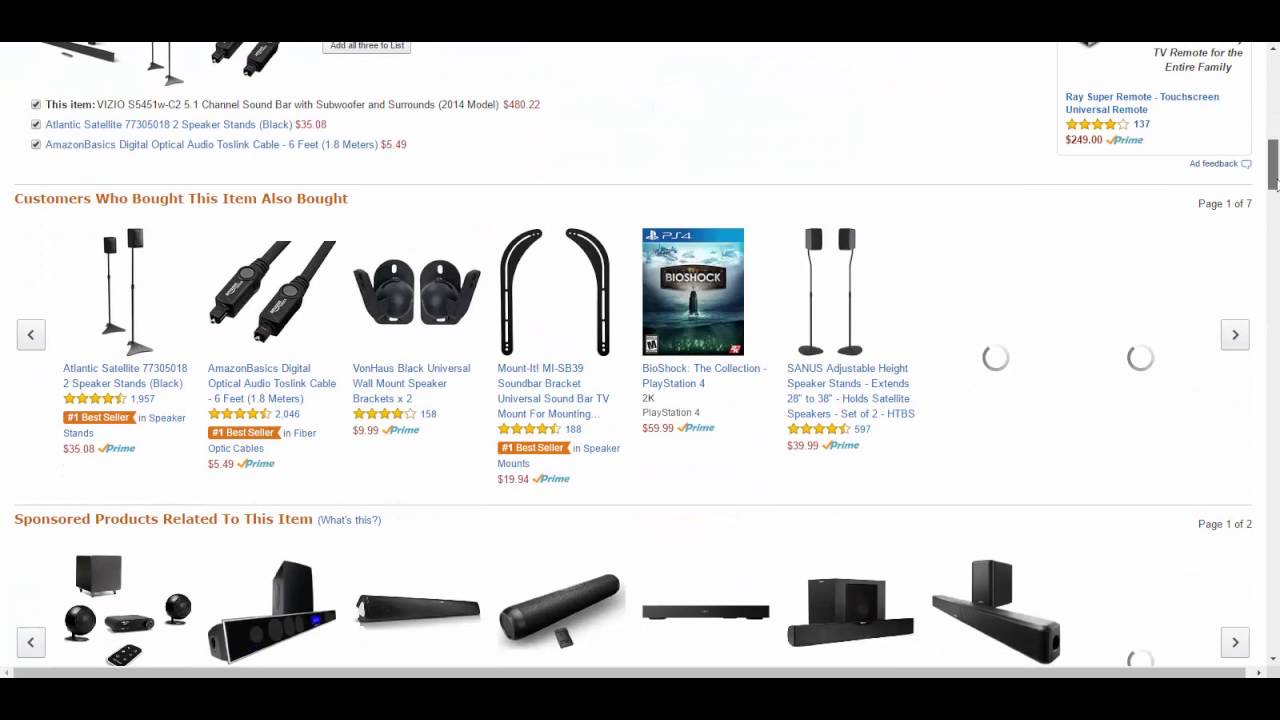This image appears to be a screenshot taken from an Amazon product page, specifically focusing on the "Customers who bought this item also bought" section. The image is zoomed in to display a variety of related items. Among the featured products are:

1. **Atlantic Satellite 2 Speaker Stands**: Clearly visible, suggesting they are popular among customers who bought the main item.
   
2. **Amazon Basics Digital Optical Audio Toslink Cable, 6 Feet**: A high-quality audio cable likely used for connecting home audio equipment.

3. **VonHaus Black Universal Wall Mount Speaker Brackets (Set of 2)**: These brackets are designed to securely mount speakers to the wall, ideal for optimizing audio setup.

4. **Mount-It Soundbar Bracket, Universal Soundbar TV Mount**: This bracket is for attaching a soundbar to a TV mount, helping to streamline home entertainment systems.

5. **Bioshock: The Collection for PlayStation 4**: A popular video game collection indicating that the main item might be related to gaming or entertainment.

6. **Satellite Speaker Mounts (Set of 2)**: These mounts are designed to hold satellite speakers, suggesting a focus on enhancing sound systems.

At the bottom of the image, there is a section labeled "Sponsored products related to this item" in orange text, with the phrase "What's this" in blue parentheses next to it. Although the descriptions of these sponsored products are not fully visible, the majority appear to be related to audio equipment, such as black speaker parts, soundbars, and computer accessories.